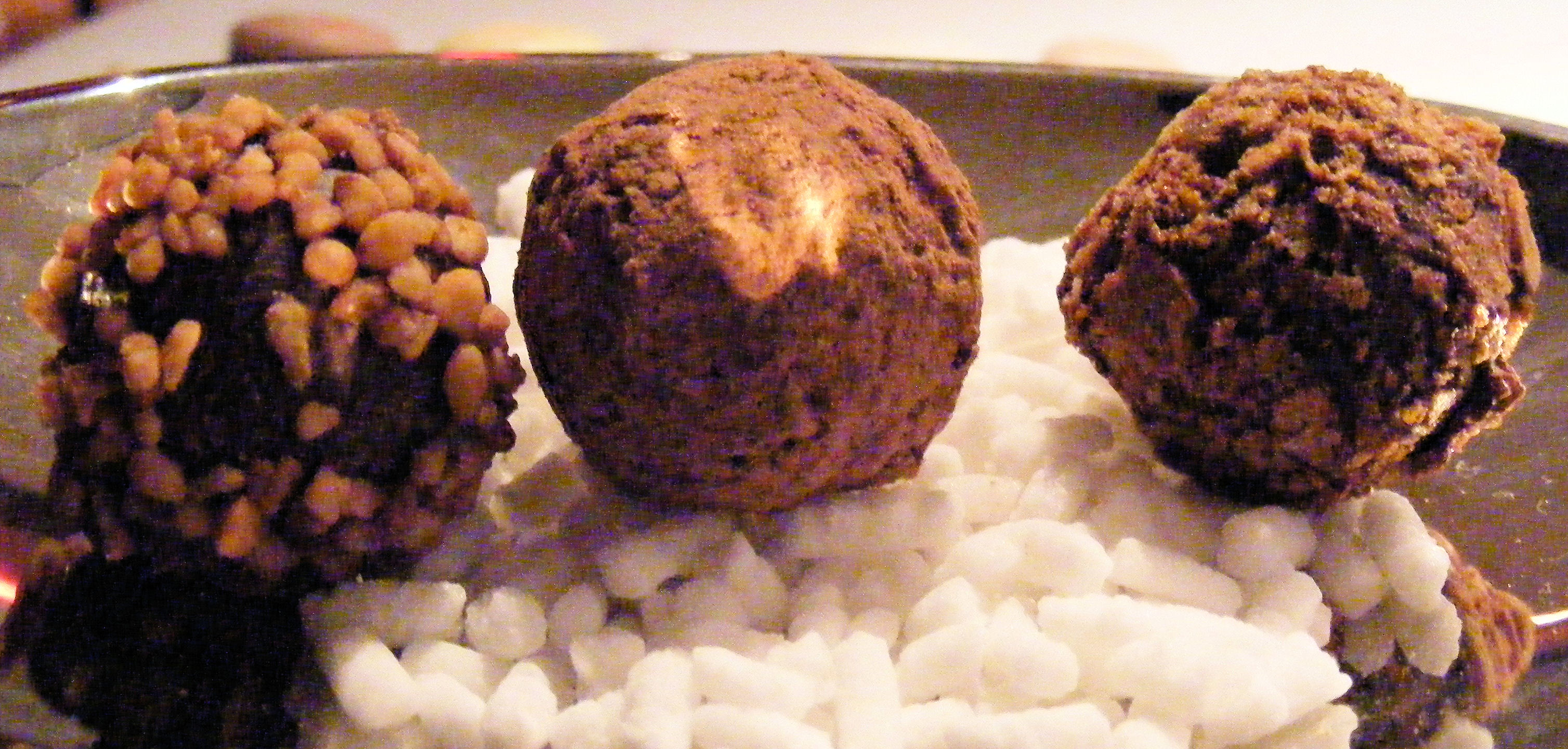The image features a close-up of three assorted chocolate truffles arranged on a round brown plate, set against an off-white background. The truffles, each with distinct toppings and textures, are nestled atop a bed of white, curd-like substance that resembles cottage cheese or another edible material. 

The truffle on the left is dark chocolate and coated with small pieces of nuts, giving it a crunchy appearance. The middle truffle is also brown but has a powdery coating that looks like cocoa powder, suggesting a rich, chocolatey flavor. The truffle on the right is dark brown as well, dusted with a slightly lighter brown powder, possibly biscuit crumbs or sugar. The picture is grainy, suggesting it might have been sourced from a magazine. The lighting highlights the textures of the truffles, enhancing their appetizing appeal.